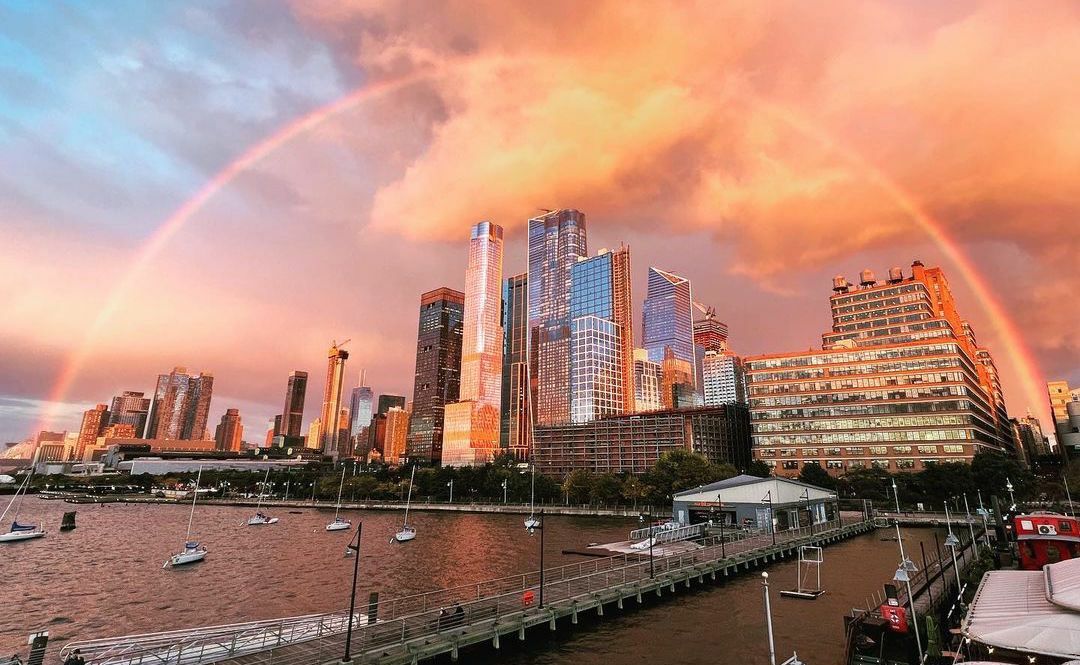This photograph captures a stunning dusk cityscape, showcasing a vibrant rainbow arching gracefully across the skyline. The city at night is bathed in hues of blue, orange, and pink, as though the sun is setting. The rainbow frames the skyline from the bottom left to the bottom right of the image. The central part of the image features a series of skyscrapers, including a cylindrical pink or orange building, a rectangular block, and a steel gray skyscraper with distinct cylindrical and rectangular sections. Additionally, there is a blue and black building with an inclined roof and an orange side, and a nearby building with a triangular roof. To the far left, there are less prominent apartment buildings and a building under construction with a crane on top. On the right, a six or seven-story steel and glass building sits beside an older structure with three water towers.

In the foreground, a bridge or walkway made of gray steel extends from the bottom left to the center of the image, leading past a one-story gray building with a gabled roof, possibly a dock for a ferry boat. This boardwalk, featuring a bench with two people sitting and some rails, forms part of a lively waterfront scene. The bottom right corner reveals another walkway and a red boat, alongside a boat with a white canvas roof. The body of water below the city holds six sailboats, identifiable by their masts but lacking sails. The image is rich in detail with lighting along the dock and a fiery hue in the clouds, creating a mesmerizing backdrop for the bustling yet serene waterfront urban night scene.